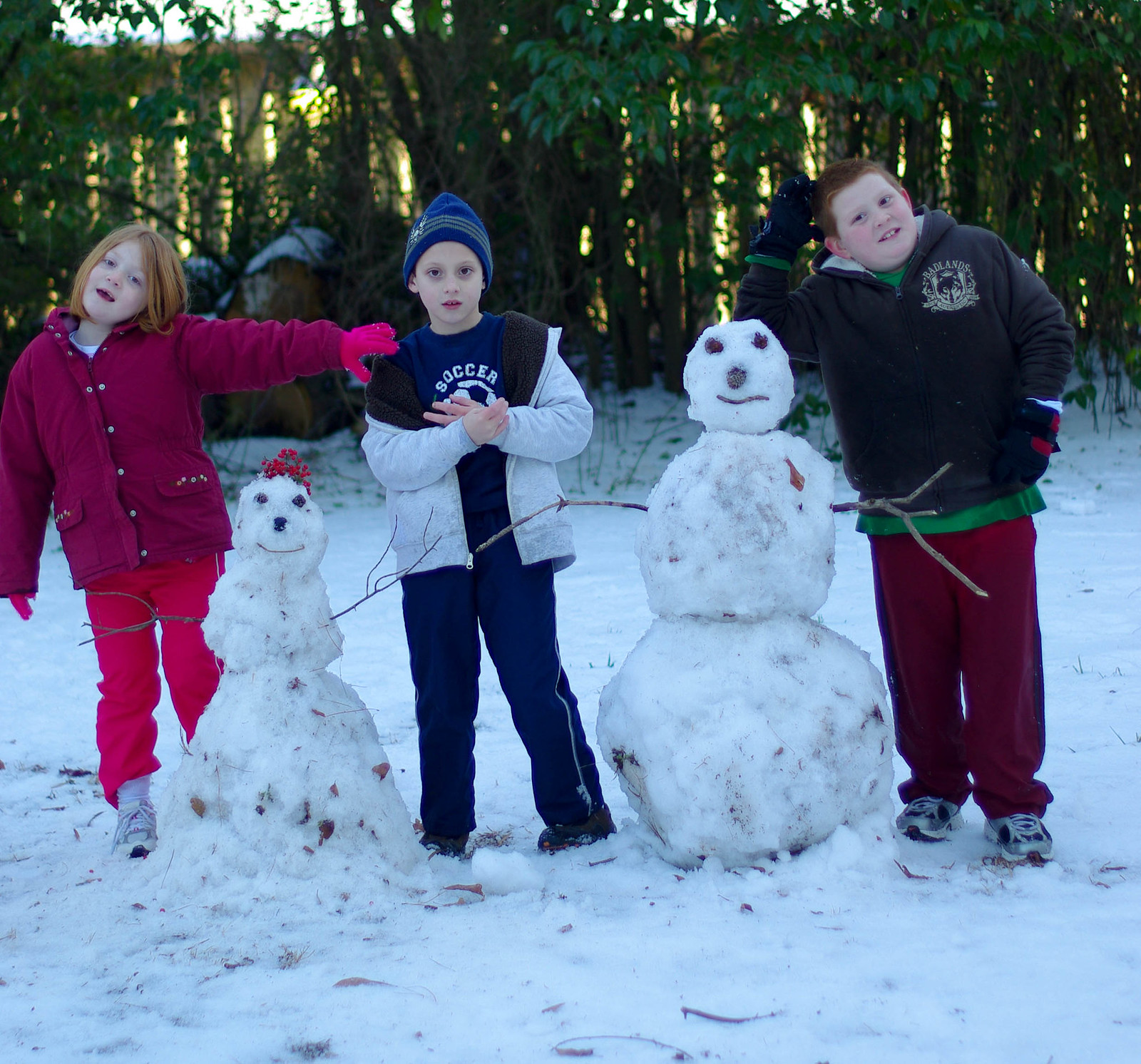In this vibrant outdoor scene, three children proudly stand beside the two snowmen they built on a thin layer of snow, with a privacy fence and trees in the background. The girl on the left, likely around 8 to 10 years old, has striking red hair and is dressed in a burgundy or magenta winter coat, hot pink gloves, and matching ski pants. She's touching the shoulder of the child in the middle, who wears a blue knit cap, an unzipped white winter jacket over a blue t-shirt that says "soccer," and blue ski pants. This middle child, whose hair is hidden by the cap, has bare hands. On the right stands a red-haired boy wearing red pants, a green t-shirt under a coat or sweatshirt, and black and red gloves. 

The children have crafted two snowmen, one short with flowers on its head, a smiley face, and stick arms, showing signs of melting with brown leaves embedded in its snow. The taller snowman, beside the boy on the right, also has branch arms, a straight stick for a mouth, and appears sturdier. Despite the sparse snow coverage of about an inch, the children’s joyful creativity is vividly captured in their snowy playground.